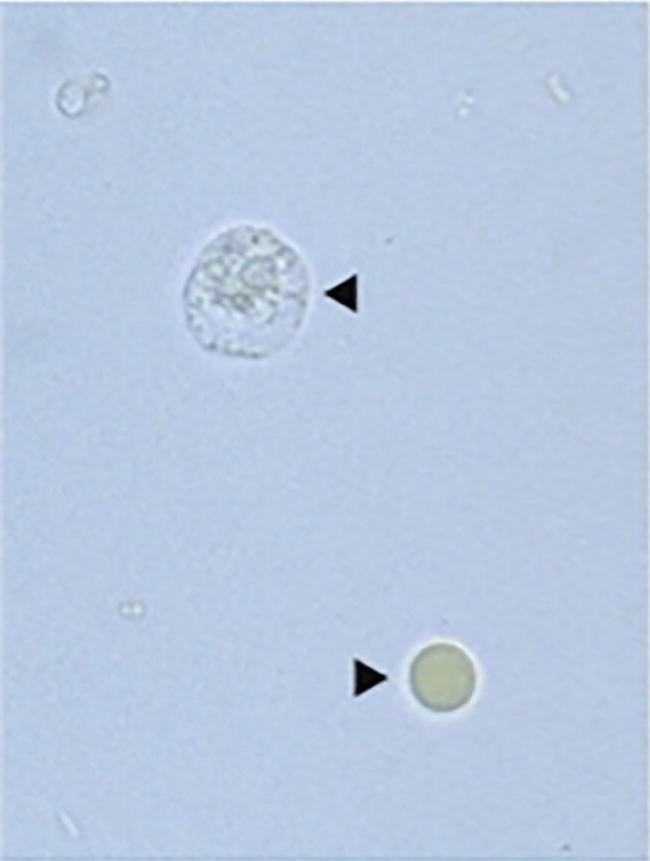The image appears to be a close-up view taken under a microscope, showcasing various microorganisms against a bluish background. In the top left portion of the image, there is a black triangle arrow pointing towards an irregular, fluid-shaped organism. Another black triangle arrow is located in the bottom right, pointing to a more rigid, circular microorganism that resembles a tiny planet. Surrounding these highlighted cells, which exhibit pale yellow and see-through crystal colors, are numerous smaller microorganisms scattered throughout the bluish gray background. The overall scene suggests a microscopic examination of cells in which these organisms are being studied.